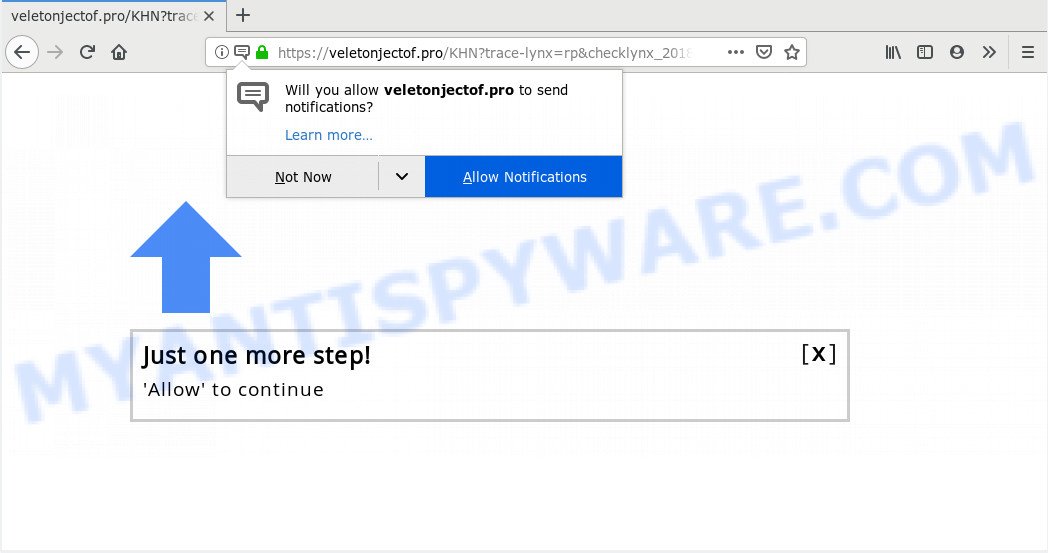Screenshot of a web browser with one tab open, displaying the address bar with the URL "veletonjecktoff.pro" prominently visible. The browser's interface includes standard navigation icons at the top. The webpage itself has a plain white background, overlaid by a diagonal watermark "myantispyware.com" in blue. Just beneath the address bar, a pop-up notification prompt is visible, asking "Will you allow veletonjecktoff.pro to send notifications?" The site name "veletonjecktoff.pro" is bolded within the prompt, and there are two interactive buttons below: a greyed-out "Not Now" button and a blue "Allow Notifications" button, separated by a down arrow. Additionally, in the lower left corner of the pop-up, a blue arrow points upward, directing attention to another box labeled "Just one more step, allow to continue." This secondary box also features a close (X) button in its upper right corner.